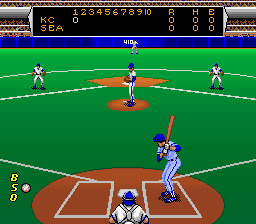In this video game screenshot of a baseball game, the perspective is from behind home plate, giving a clear view of the game in progress. The catcher is crouched down in a ready position, fully focused on the pitcher who is preparing to throw the next pitch. The batter, adorned in a white uniform with a blue jersey underneath and a matching blue baseball hat, stands alert at the plate, eyes fixed on the pitcher. 

On the field, a player is positioned between first and second base, while another stands between second and third base, both in identical uniforms as the batter and catcher. In the background, the scoreboard is visible, displaying the team abbreviations "KC" and "SEA." The score indicates that it is still the first inning, with KC yet to score, and SEA currently at bat. This detailed setting captures the tense moment just before the pitch is thrown, reflecting the realistic and immersive nature of the video game.